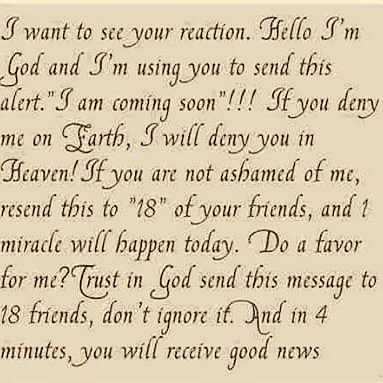The image is a tan square piece of paper entirely covered with a curvy, distinct text. This text prominently displays a chain message designed for social media, urging the recipient to spread it to 18 friends. The message reads: "I want to see your reaction. Hello, I'm God, and I'm using you to send this alert. I am coming soon!!! If you deny me on earth, I will deny you in heaven! If you are not ashamed of me, resend this to 18 of your friends. One miracle will happen today. Do a favor for me: trust in God, send this message to 18 friends, don't ignore it. In 4 minutes, you will receive good news." The entire message is written in tan and brown colors and exemplifies a typical superstitious chain letter.